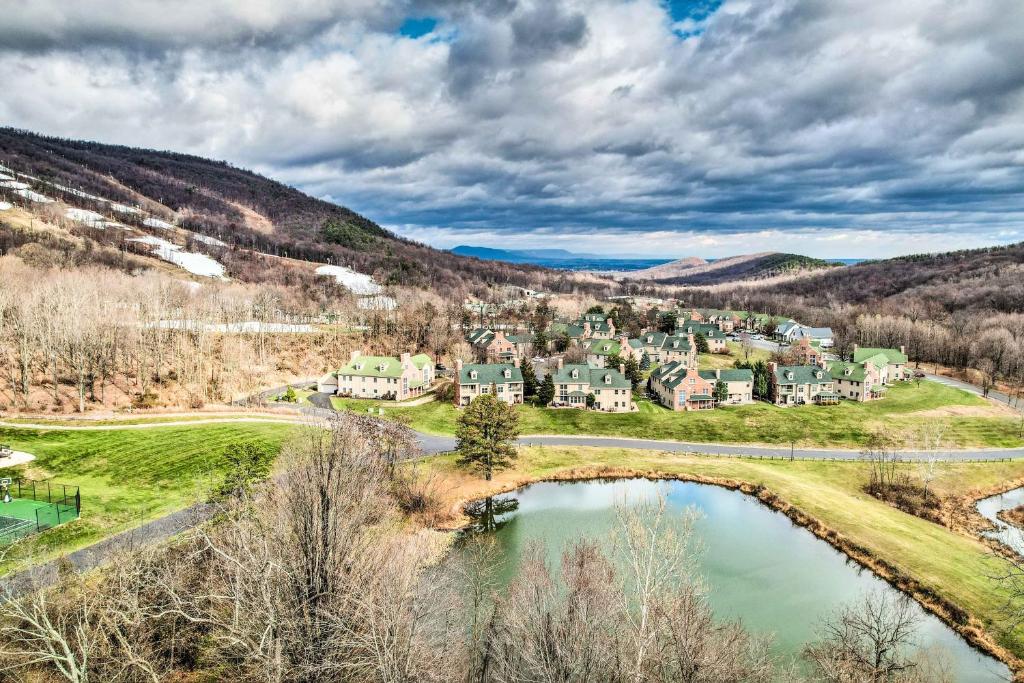This detailed landscape painting captures a cloudy day with a dynamic sky featuring both white and dark clouds against a bright blue backdrop. In the center-left portion of the image, a higher hill adorned with grass dominates the skyline, while a series of brown hills extends to the horizon, adding textural depth to the scene. Nestled between these hills is a large village, comprised of around a dozen buildings. The buildings are notable for their distinct green roofs in varying shades of light and dark green. A road meanders in front of the village, bridging the gap between the hills and the foreground. In the immediate foreground, a substantial, oval-shaped lake is encircled by grassy fields and trees, which are notably barren, suggesting an autumn or winter setting. Additionally, tree branches stretch across the lower section of the painting, framing the serene waters of the lake, which appear to be a communal spot for the village inhabitants. Overall, the painting evokes a sense of tranquility amidst a slightly turbulent weather, with potential hints of rain and distant thunder.